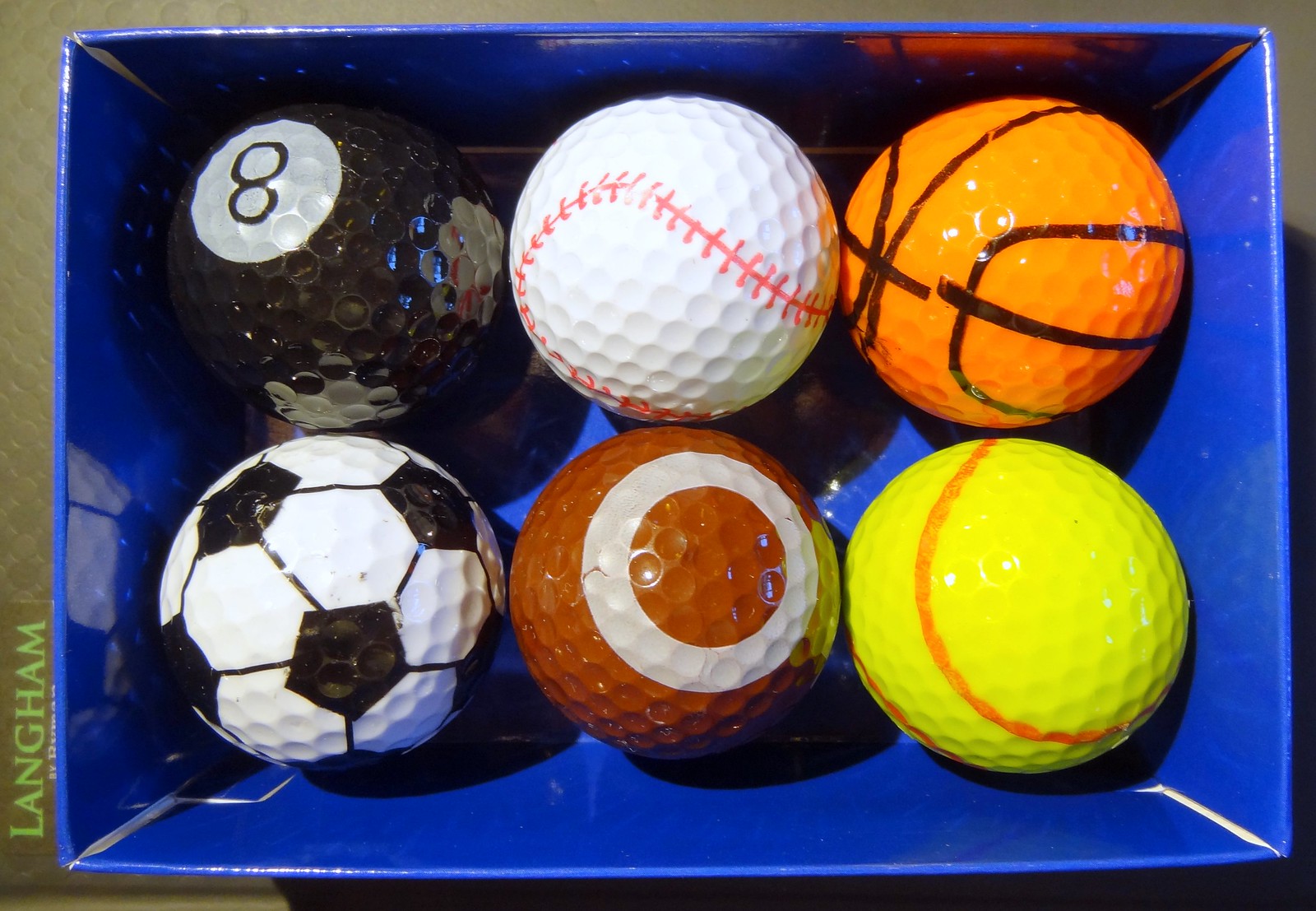The image depicts an overhead view of a glossy blue box containing six golf balls, each cleverly decorated to resemble a different type of sports ball. The golf balls are arranged in two neat rows of three inside the bright blue box. 

- **Top Row (from left to right)**:
  - A black golf ball resembling an eight ball from billiards, complete with a white circle and the number 8.
  - A white golf ball painted with red stitching to mimic a baseball.
  - An orange golf ball featuring brown lines to look like a basketball.

- **Bottom Row (from left to right)**:
  - A white golf ball with black patterns resembling a soccer ball.
  - A brown golf ball with a white circle on one tip, designed to look like a football.
  - A bright yellow golf ball with red stripes at each end, imitating a tennis ball.

On the left-hand side of the box, the word "LANGHAM" is written vertically in a green serif font in all capital letters. The photo, possibly a product image, is taken on a concrete surface, providing a muted backdrop that makes the blue box and colorful golf balls stand out vividly. The detailed decoration of each golf ball accentuates their distinctive designs, emphasizing the novelty and uniqueness of the set.